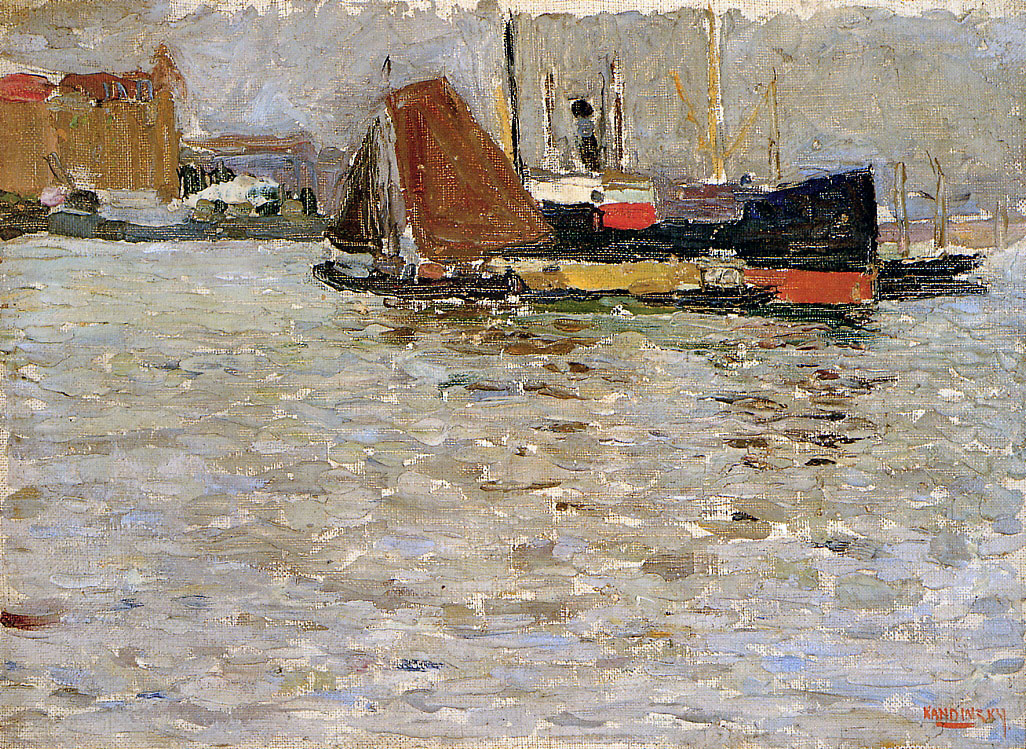The painting appears to be an oil on canvas, possibly done in an expressionist style, and depicts a harbor scene with a blend of muted and vibrant colors. The composition is somewhat blurred, giving it a vague and hazy appearance. The central focus includes a large black boat with a yellow and red bottom, alongside a small sailboat with a brown sail. The water surrounding the boats features earthy greens, blues, and grays with visible waves, reflecting the sky above, which is painted in dark gray. On the left side of the painting, there are tan rectangular buildings with red roofs situated by the dock, with cranes positioned below and in front of them. In the distance, another black boat is visible near these buildings. The painting captures the essence of a bustling harbor through its use of diverse colors and slightly distorted forms, adding a unique depth and movement to the scene.